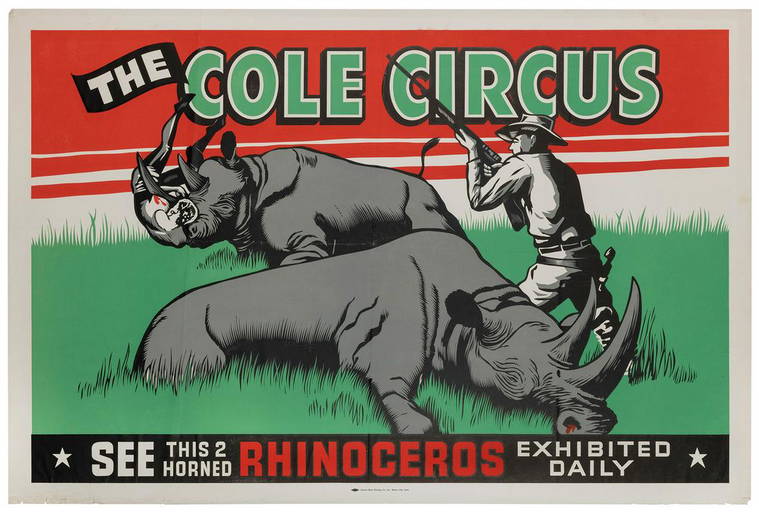This detailed poster for the "Kohl Circus" features a vivid color illustration bordered in gray. Dominating the top portion is a red banner with a smaller black banner inside it. The black banner displays the word "THE" in white text, while "Kohl Circus" is written below in stylized green letters outlined in white and black. Centered in the image are two rhinoceroses depicted in a high grassy field. One rhinoceros lies on the ground with blood streaming from its nostril, while the other appears to be in the process of falling, presumably shot by a hunter. The hunter, standing to the right, wears light-colored clothes, a cowboy hat, and holster, and holds a rifle aimed at the rhinoceros. This dramatic scene is rendered in a hand-drawn style that might be computer-animated as well. At the bottom of the poster, a black banner features white text and two stars, one on each end, reading: "SEE THIS TWO-HORNED RHINOCEROS EXHIBITED DAILY."